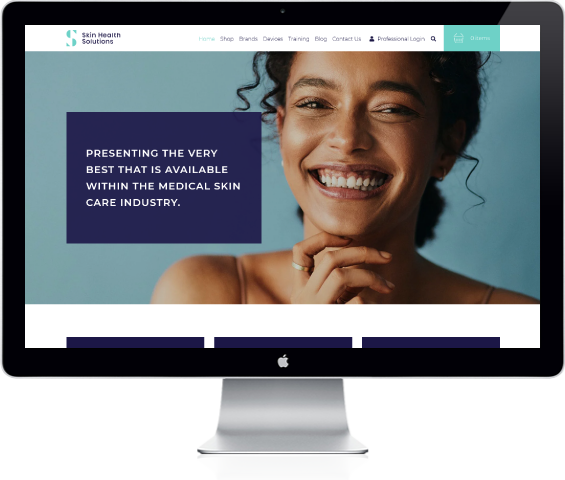The image depicts a flat-screen monitor displaying a website interface. The monitor's stand, made of brushed aluminum, features a modern, curved design. The screen shows a website for "Datton STAIN Health Solutions," with navigation options for Home, Shop, Brands, Devices, Training, Blog, Contact Us, and Professional Login. There is an indication of zero items in the cart. Despite the overall fuzziness and poor resolution, the elements are somewhat recognizable.

On the screen, there's an image of a young woman, possibly of African descent, with bright white teeth and visible gums, laughing. She has her hair styled in a low bun at the back of her neck. Beside her image, a blue box presents a message in white font: "Presenting the very best available within the medical skincare industry." The background behind her is turquoise, contrasting with the dark blue of the message box.

At the bottom edge of the screen, the distinctive white Apple logo is visible, hinting that this is an Apple monitor.